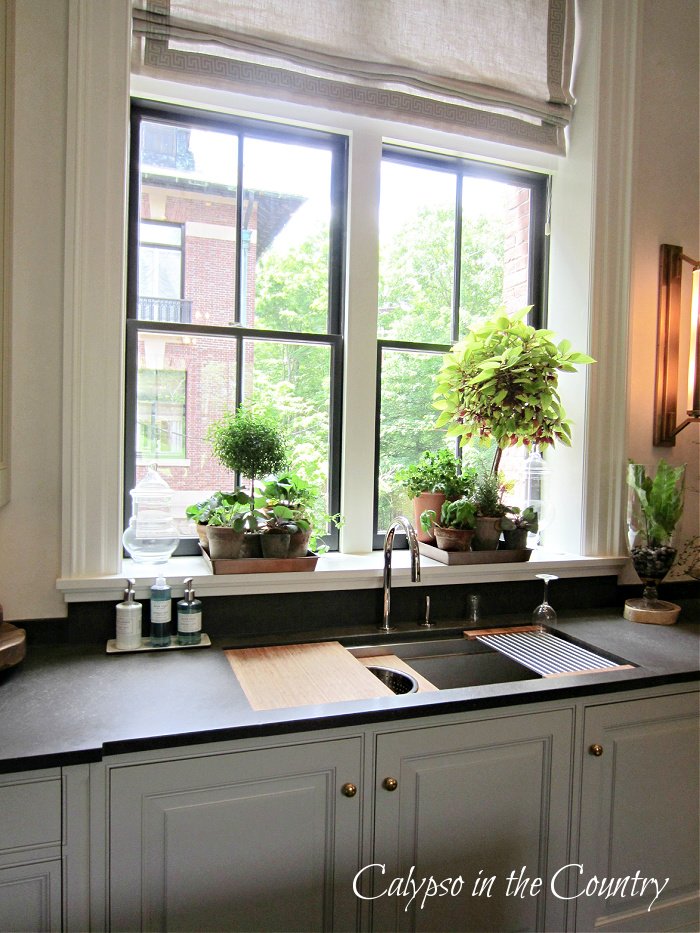This detailed photo captures the charming interior of a bright, sunny kitchen, centering around a stainless steel sink situated beneath a large double window with four panes on each side. The windowsills host a vibrant array of nearly a dozen small plants, varying from leafy greens to shrubby, tree-like plants, all set in an assortment of small pots and trays. Outside the window, a lush green tree stands next to a visible brick building. The countertop is black with a matte finish and features a variety of items: on the left side, three small bottles of hand soap rest on a silver tray near a wooden cutting board, while on the right side, there's another small green plant that resembles a cactus, perhaps growing in a bottle, and several rods that might be for drying dishes. The scene is illuminated with natural light, enhancing the pristine, cozy appeal of the white cabinets below the sink. A subtle textual overlay at the bottom of the photo reads "Calypso in the Country," contributing to the serene and inviting ambiance of this homey kitchen setup.